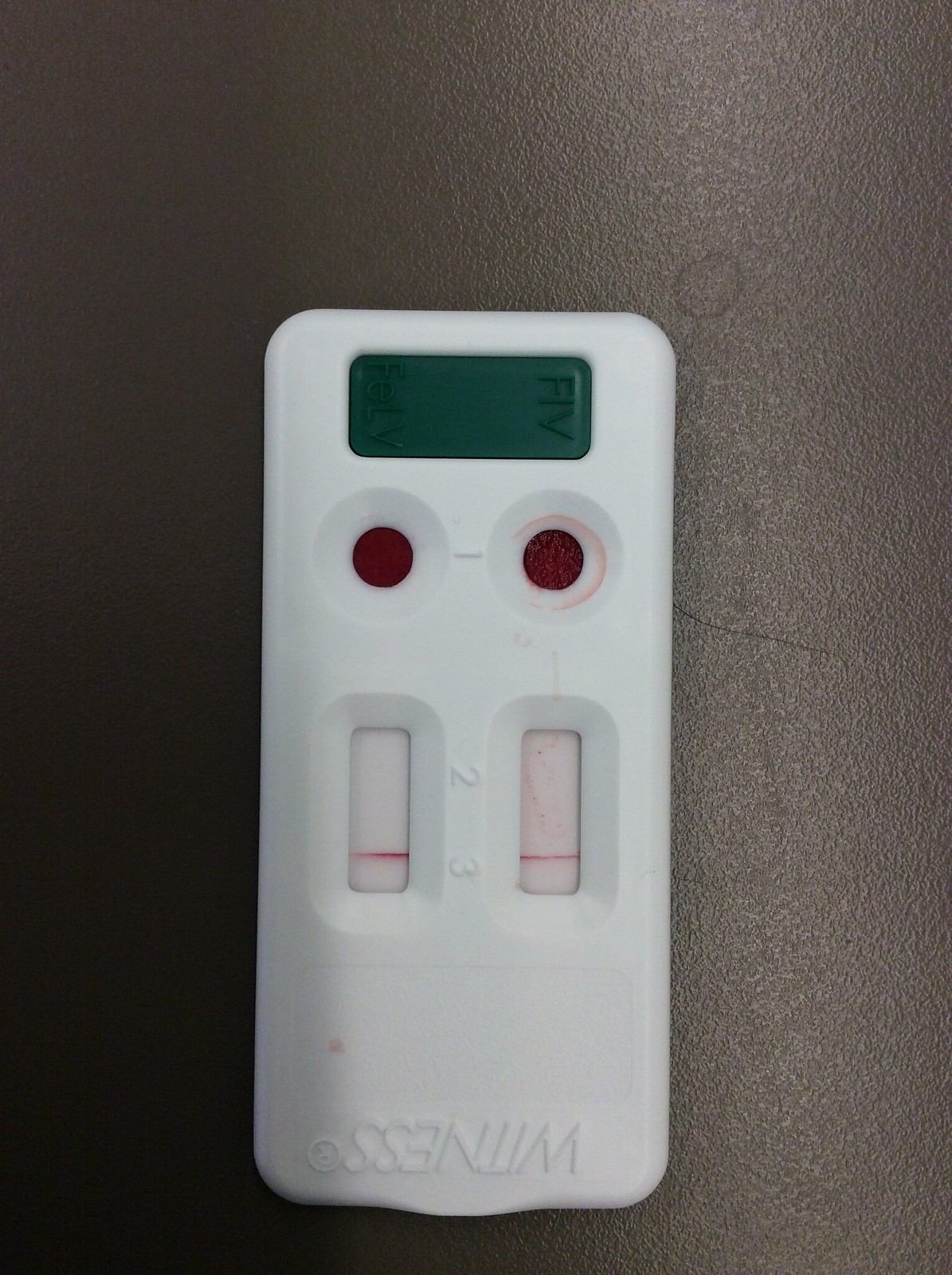The image features a close-up of a white plastic test cartridge, presumably a diagnostic device like a pregnancy or another type of urine test. The cartridge is positioned on a black, grainy surface, likely a tabletop. The word "Witness," accompanied by a trademark icon, is printed across the top of the cartridge. The middle section contains two rectangular depressions, each displaying a faint pink line, separated by the numbers "2" and "3". Further up, there are two circular depressions, also appearing to contain test result indicators, with the number "1" situated between them. At the far end of the cartridge is a rectangular digital display with a gray background showing the letters "FIV." The detailed features of the cartridge and the results indicate a comprehensive diagnostic test layout.